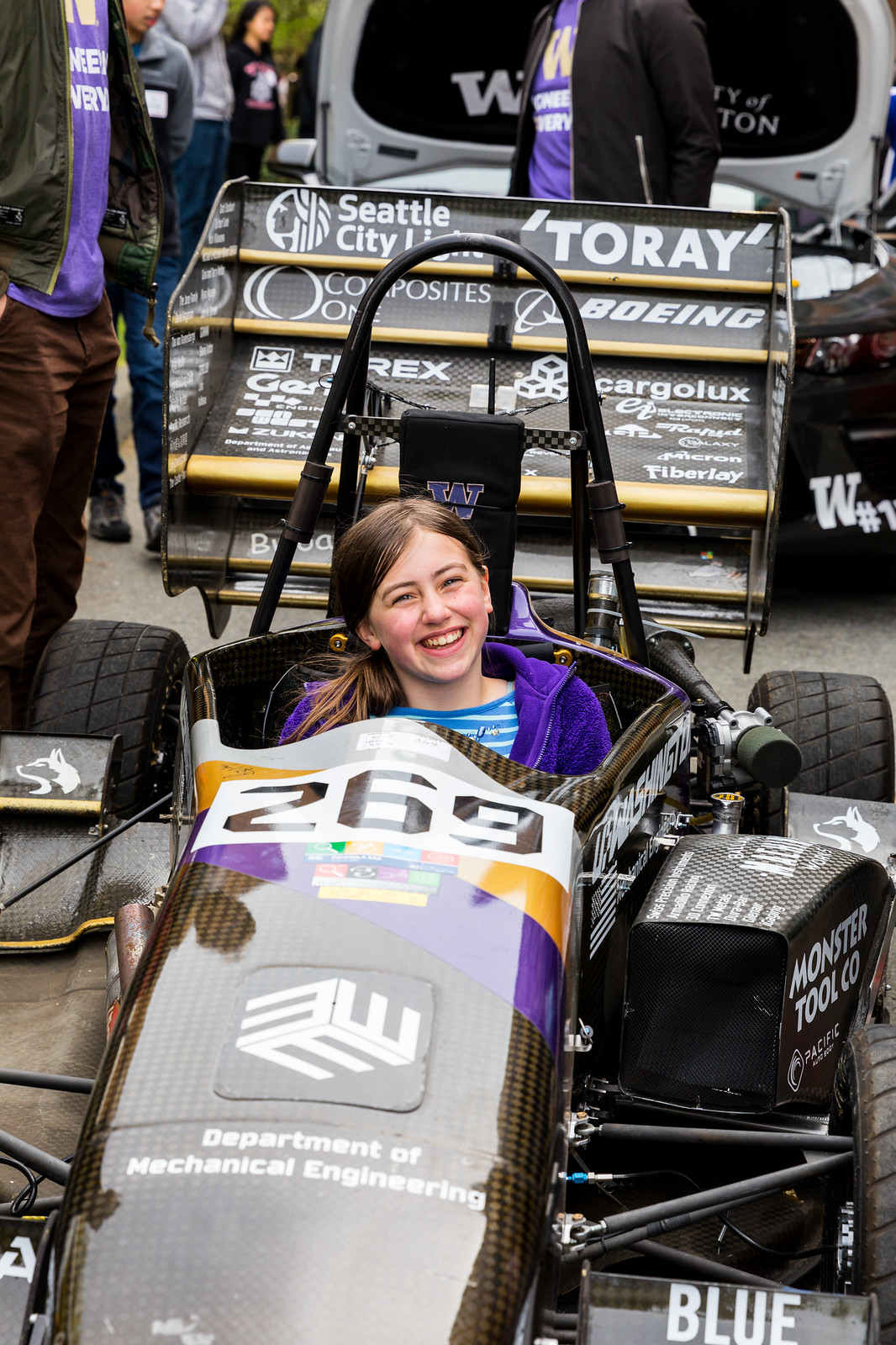In this vibrant outdoor photograph, a young girl with long brown hair swept to the side is beaming at the camera as she sits inside a sleek, homemade race car numbered 269. This impressive vehicle, predominantly black with purple and yellow accents, proudly displays "Department of Mechanical Engineering" at the front. The girl's attire includes a blue and white striped shirt paired with a purplish jacket, adding a splash of color to the scene. Behind her, there's a display featuring names of several businesses, including partially obscured "Seattle City", Boeing, Tyrex, and Cargolux. Surrounding the main focus are various elements that suggest a car event or show: a vehicle with its hood up displaying the engine, people clad in sweatshirts and blue shirts, and large tires to the girl's left. A man, wearing a purple t-shirt, green or black jacket, and burgundy slacks, stands nearby with his hands in his pockets, partially cropped out of the photo. The clean and detailed composition brings to life not just the girl's joy but the bustling atmosphere of this car-centric gathering.